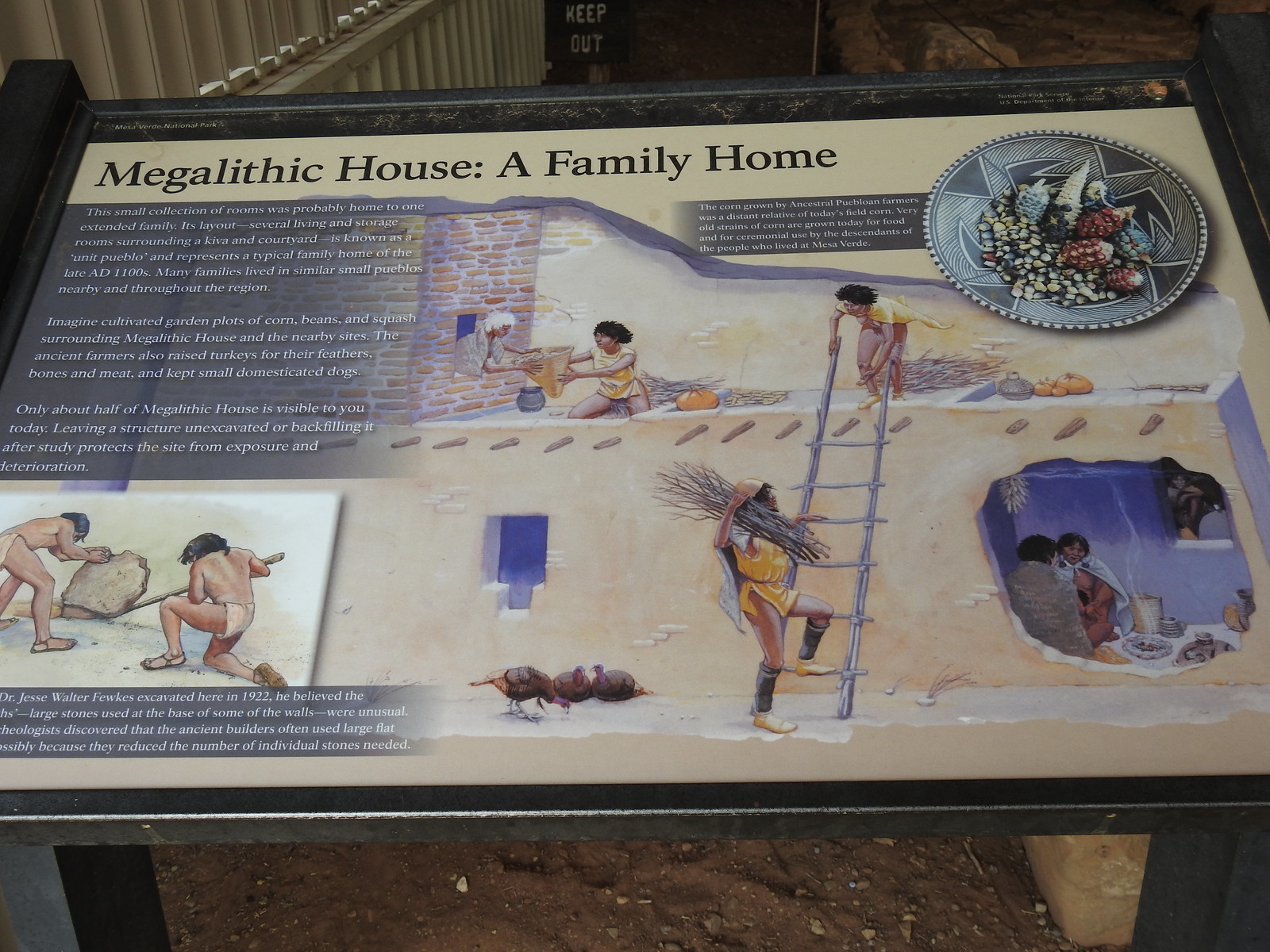The image captures a detailed museum exhibit featuring a rectangular informational sign encased in a black-bordered frame with a clear plastic cover. The sign provides comprehensive information about megalithic housing. At the top, it reads “Megalithic House, a Family Home” against a tan background with black text. 

Central to the sign is an illustration depicting a scene from megalithic times, illustrating a family living in a megalithic house. The house has tan walls and a red brick chimney. A wooden ladder leans against the house, with a man preparing to climb it while carrying a bundle of sticks. A child stands at the top of the ladder on an upper floor, and a woman is kneeling next to the stone chimney, handing a basket filled with food to someone leaning out of the chimney. 

The right side of the illustration presents additional elements: ancestral farmers growing corn, a tribal dish with corn, small chickens, and people using tools inside the stone homes. In the background, the scene has a dirt floor and a small, white fence with a "Keep Out" sign posted above it in the top left corner. Text on the left-hand side of the sign explains the significance of these illustrations, providing context to the megalithic family's daily life and their agricultural practices.